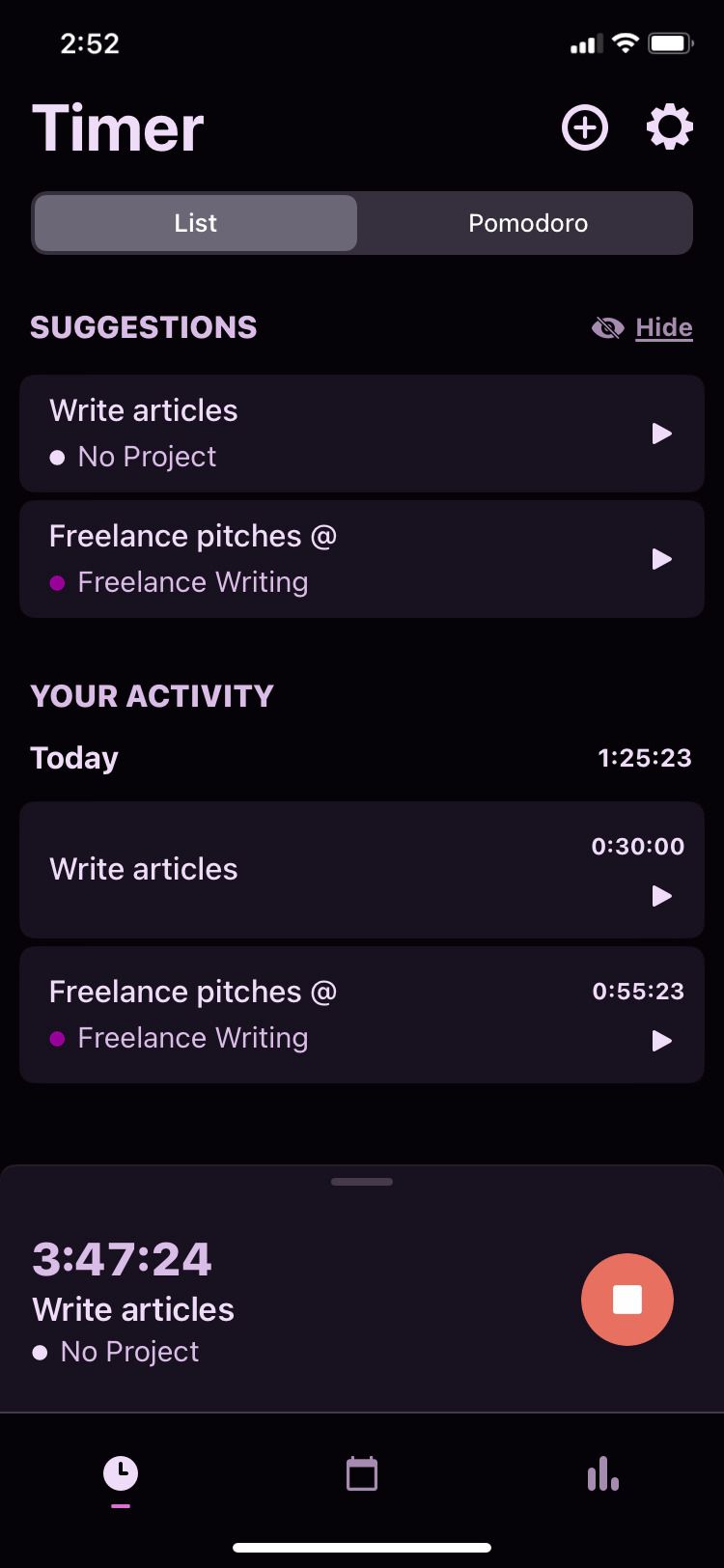The image displays a smartphone screen showcasing a productivity app. At the top-left corner, the time reads 2:52. On the top-right corner, indicators for signal strength, Wi-Fi connection, and battery life are visible. Beneath this, on the left side in large font, is the word "Timer". To its right, there is a circle with a plus sign and a small cogwheel icon, likely for adding tasks and accessing settings, respectively.

Directly below is a grey strip bifurcated into two sections: one light grey labeled "List" and the other dark grey labeled "Pomodoro". Under this strip, the word "Suggestions" appears on the left-hand side, followed by two dark grey panels. The first panel reads "Write Articles" with a bullet point labeled "No Project" in yellow. The second panel reads "Freelance Pitches" with a bullet point labeled "Freelance Writing" in purple.

Further down, there is a section titled "Your Activity Today". Underneath, two grey panels identical to the previous ones are listed, but the "Write Articles" panel lacks the "No Project" subtext. Both panels display time durations on the right-hand side: "Write Articles" shows "03:00:00" and "Freelance Pitches" shows "05:55:23".

At the very bottom of the screen, a final panel mentions "34:47:24 Write Articles" with a bullet point labeled "No Project". A red circle with a white square in the center is positioned on the right side of this panel.

This detailed display suggests a focus on time management tasks, integrating elements of the Pomodoro technique and task categorization for improved productivity.